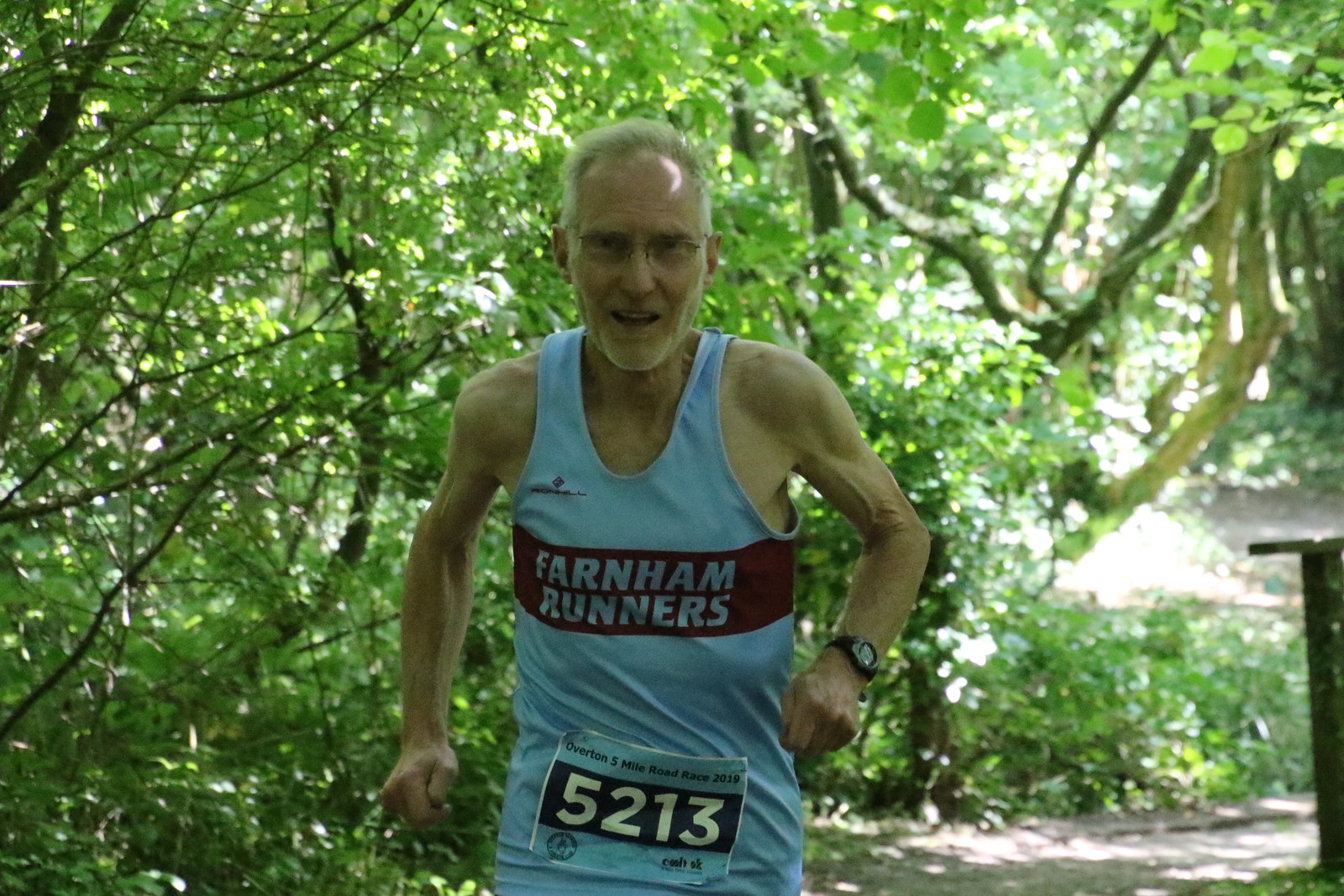The photograph captures an older gentleman, likely in his 60s, actively running towards the camera on a trail or road, possibly in the middle of a marathon. He has short-cropped white hair, a light complexion, and is slightly balding with a touch of grey stubble. Sporting glasses, he wears a blue and dark red tank top that reads "Farnham Runners" with the number 5213 taped to the front. His physique is both muscular and lean, suggesting a dedicated runner's build. Despite the exertion, he wears an open-mouthed smile. The background features abundant trees and foliage, indicative of a park setting. The bright natural sunlight bathes the entire scene, creating a vivid, well-lit outdoor environment. There are no other individuals in the image, focusing the attention solely on the determined runner.